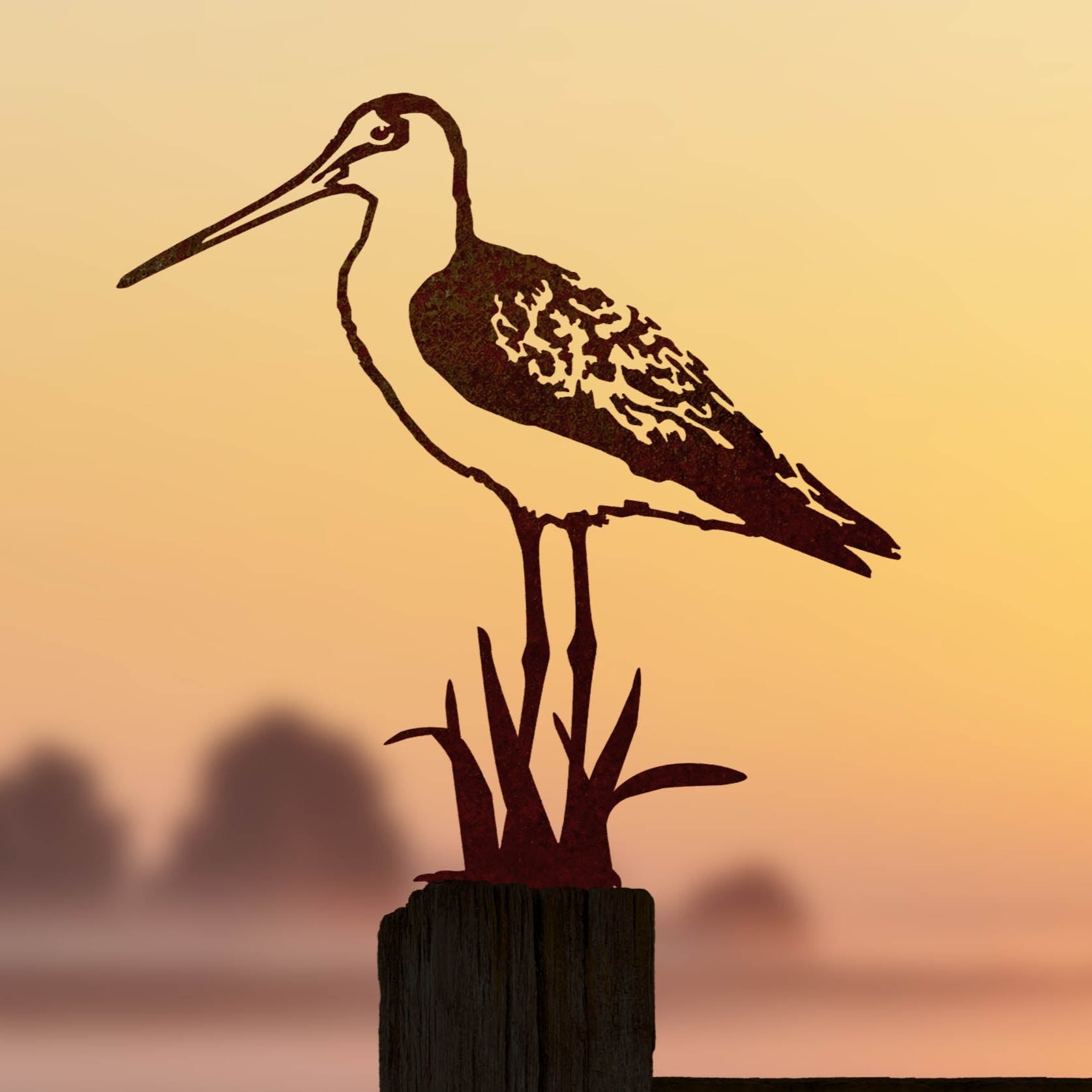An illustrated, square-shaped image features a surreal sky with a gradient transition from golden hues at the top to pink tones at the bottom. The background is artistically blurred, creating an impression of distant hills bathed in soft, abstract colors. Superimposed prominently on this backdrop is a simplistic yet expressive drawing of a seabird, possibly a gull. The bird, depicted with minimalistic brush strokes, is characterized by its small bill, a single visible eye, a white body, and feathers detailed in shades of brown and white. This charming seabird is perched atop a pole, suggesting a scene set near a pier. The overall composition combines dreamy atmospheric elements with whimsical artistry.